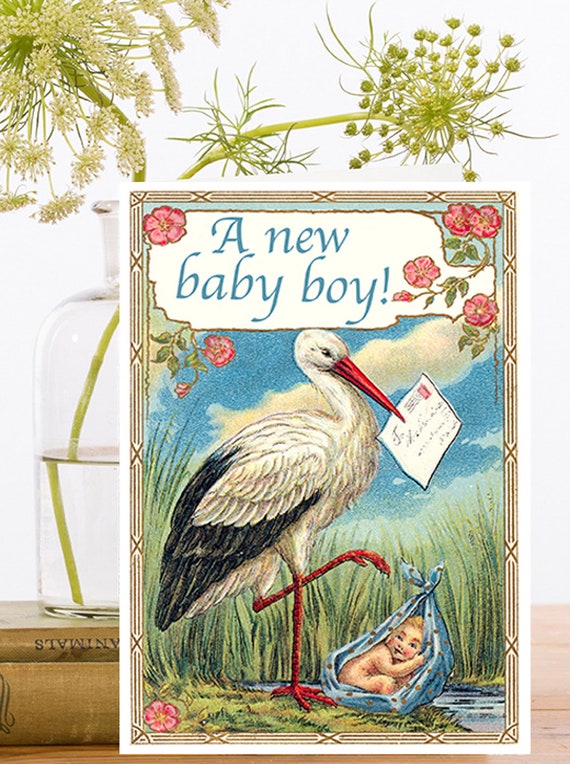The photo showcases a charming greeting card celebrating a new baby boy, placed on a wooden table. The card features a white stork with black tail feathers, orange legs, and an orange beak, standing on one leg and holding a letter with a stamp and address in its beak. Below the stork, a baby wrapped in a blue, dotted blanket with rosy cheeks rests on the ground, surrounded by marshy grass. The card's edges are adorned with a gold, old-fashioned bamboo print border and accented with hibiscus flowers in three corners. In the background, a blue sky with a feathery cloud adds to the picturesque scene. Behind the card, a clear vase half-filled with water holds a single green flower stem, creating a delicate contrast. The vase sits atop two stacked books, adding an element of rustic charm to the composition. The backdrop of the photo is white, and the scene is brightly lit, highlighting every intricate detail.